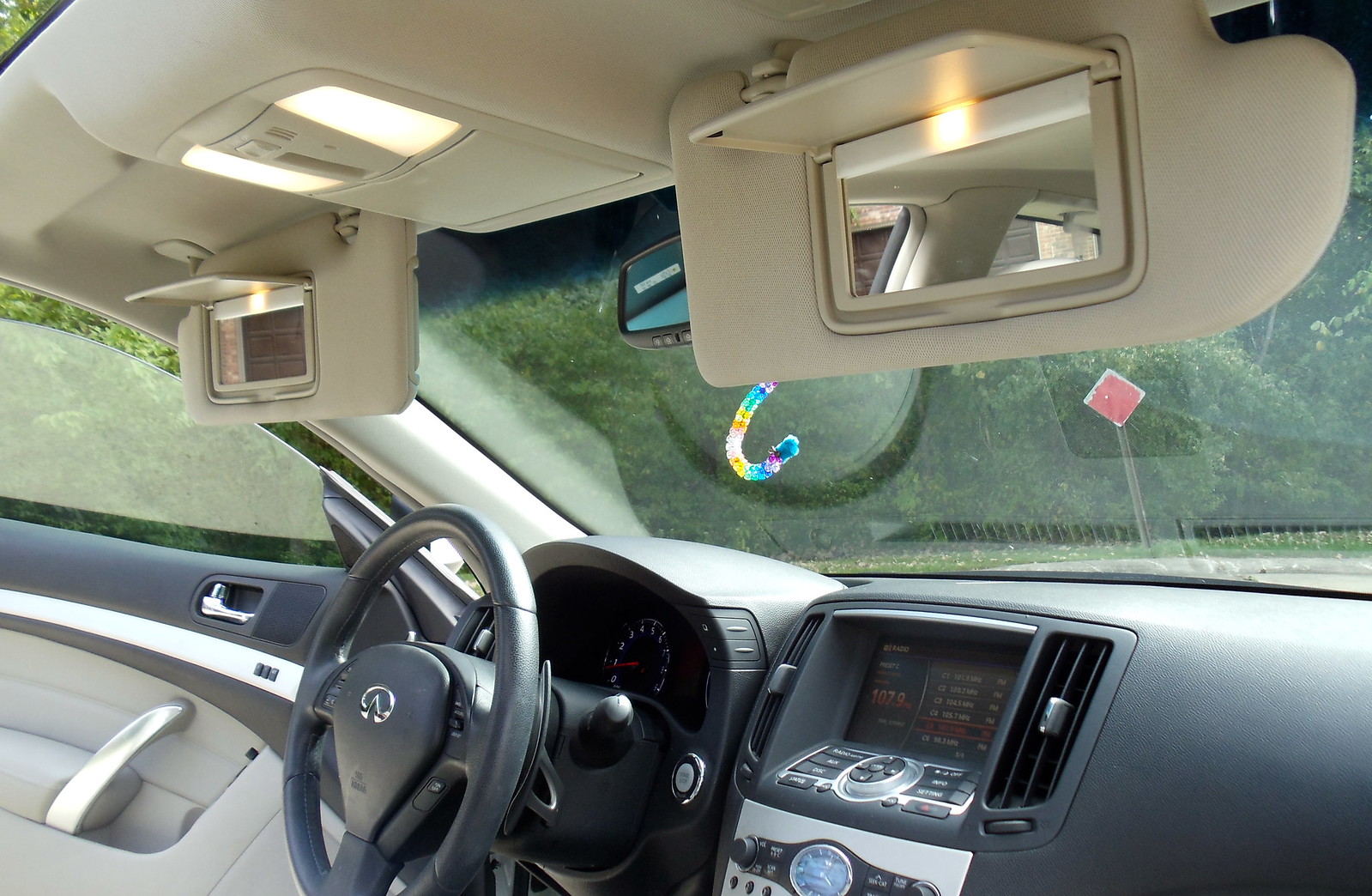This detailed color photograph captures the inside of a car, viewed from the passenger seat. The dashboard is predominantly black, including a central electronic screen with buttons and a round knob below it. Both sun visors are flipped down, and their mirrors are opened with lights turned on. The vehicle's make is identifiable by the silver emblem on the black steering wheel, resembling an infinity symbol. The interior features black leather, contrasting with a light gray lower door panel and a tan-colored roof. The driver's side door is open, revealing a partially beaded chenille stick hanging off the rearview mirror, intricately decorated in blue, yellow, green, and white beads. Outside, trees and grass can be seen through the open door. The image is well-lit, emphasizing both the features inside the car and the natural scenery beyond.